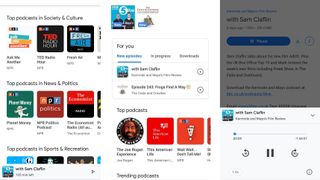The image appears to be a screenshot of a media or content dashboard, divided into three main sections. 

The left section features a variety of categories including "Top Picks in News and Politics" and "Top Picks in Sports and Recreation", along with suggestions, though the text is too small to decipher.

The middle section highlights a personalized area labeled "For You". Below this heading, there is a section titled "Top Podcasts", displaying clickable logos for various podcasts. At the bottom of this section, there is mention of "something spending, something podcasts".

The right section has a gray overlay partially obscuring the content but presents the text "with Sam Claffin". Below this, there is a blue button. Additionally, there are navigational controls in a white section at the bottom: a left-facing refresh arrow, a pause button, and a right-facing refresh arrow.

Overall, the dashboard presents curated content across multiple categories and interactive features for navigating and accessing media.